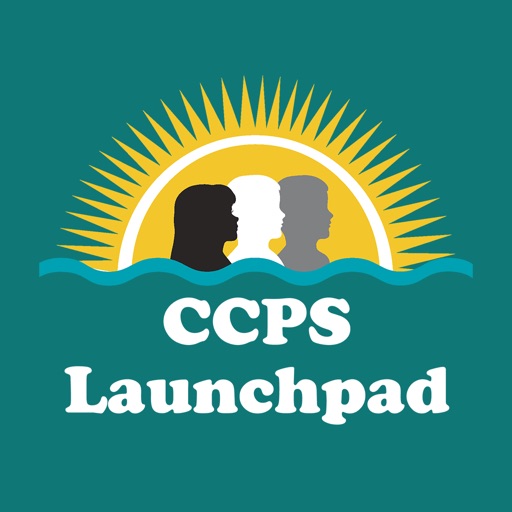The image is a square poster or note card, possibly serving as a logo or cover for a product like a CD. The background is a dark greenish hue, creating a visually striking backdrop. Dominating the lower section of the image are large, white uppercase letters spelling "CCPS," with "Launchpad" in slightly smaller font directly below. A wavy, lighter green line runs horizontally above the text. The upper portion features a graphic of a sun, depicted as a gold semi-circle with a white band encircling it and gold rays extending outward. In front of this radiant sun are three silhouetted profiles: one black, one white, and one gray. These profiles range from dark to light and suggest the inclusion of diverse individuals. This striking design is likely part of the branding for CCPS Launchpad, a cloud desktop that provides access to school resources from any location.